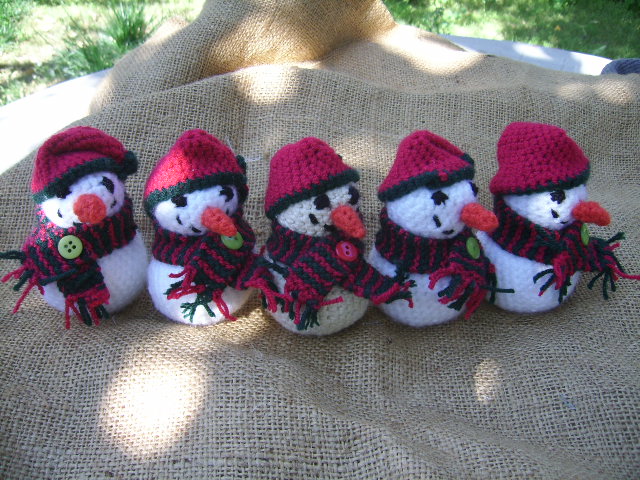In a sunlit outdoor scene, the image features a textured burlap fabric spread over a grassy background, with patches of green and brown grass peeking through. The sunlight creates varied shadows and highlights on both the grass and the burlap material, giving the latter a somewhat gray appearance with hints of tan where the light strikes. Resting atop this burlap are five intricately crocheted snowmen. These snowmen are dressed uniformly, each sporting a red hat trimmed in black with a black pom-pom on top. Their faces are adorned with black eyes and distinctive carrot-shaped noses, with parts of their smiles visible. They are also outfitted with black and white scarves. Most snowmen have green buttons on their white bodies, except for the one in the middle, which has a red button. The positioning of these snowmen varies, with the first facing forward and the others shown in profile. The entire arrangement rests casually on the wrinkled burlap, adding to the charm of the handcrafted scene.